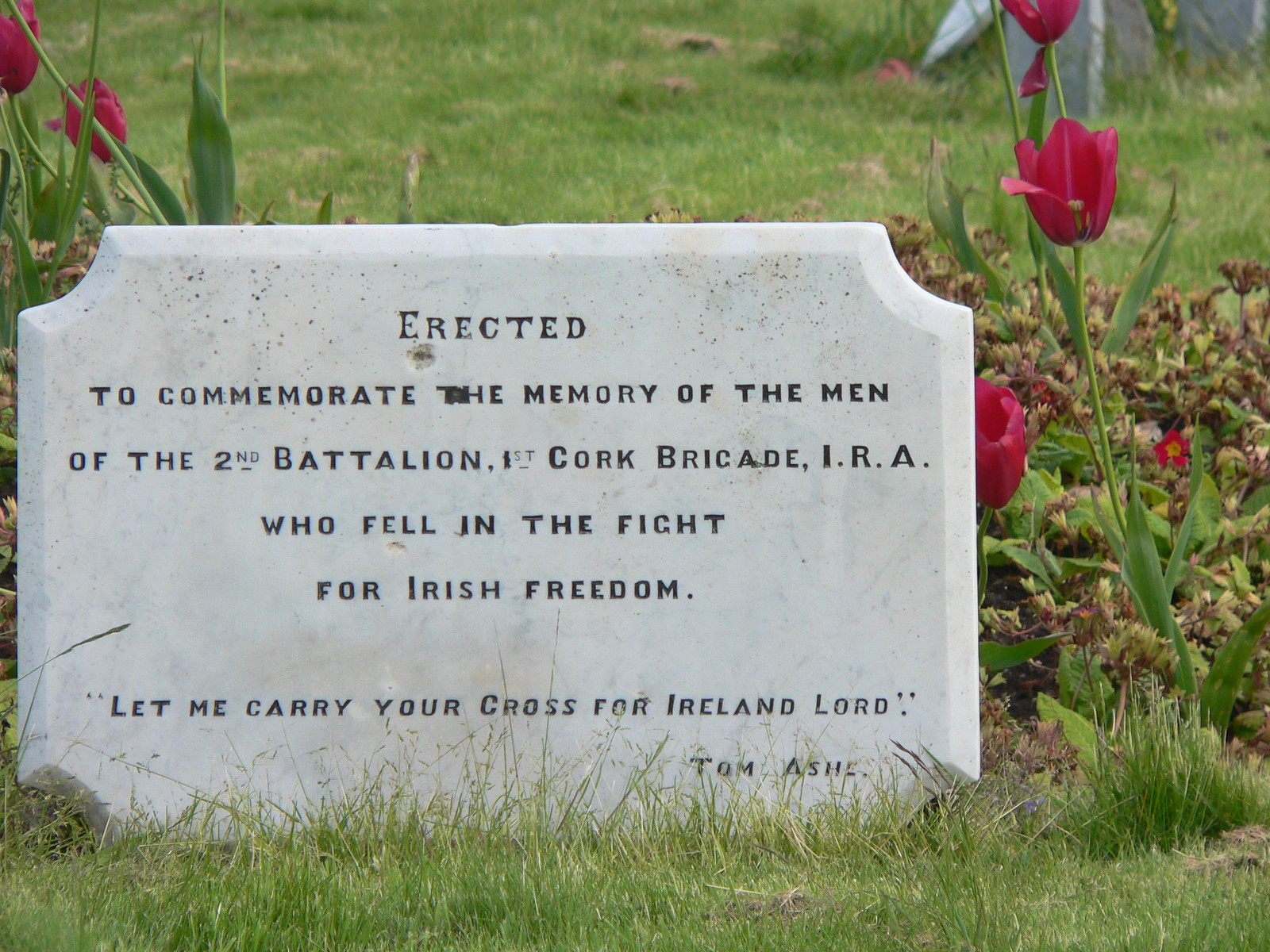In the image, there is a rectangular stone memorial with concave indentations at the corners. This light-colored plaque is engraved with the dedication: "Erected to commemorate the memory of the men of the 2nd Battalion, 1st Cork Brigade, IRA, who fell in the fight for Irish freedom." At the bottom, it features a quote in black: "Let me carry your cross for Ireland, Lord," attributed to Tom Ash. The memorial stands upright in the middle of a slightly overgrown flower bed, surrounded by faded grass that appears to have been mowed some time ago, leaving clumps of dried grass. Red tulips bloom around the monument, with about three on the right side and two on the left side. Behind the memorial, there are some brownish-green weeds or plants, adding to the slightly untidy yet poignant setting.